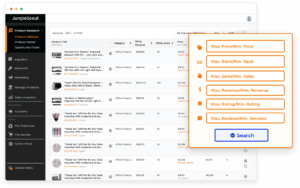This is an extremely blurry screenshot from an unidentified webpage. The illegible writing on the page obscures any informative content. The left side features a black vertical bar with indiscernible text, adjacent to a white window also containing unreadable writing. A prominently white pop-up window, outlined in orange and filled with orange text, overlays part of the page. At the very bottom, a blue bar is visible with the word "search" written on it. The image contains no photographic elements, people, animals, plants, flowers, trees, buildings, man-made structures, automobiles, helicopters, airplanes, bicycles, boats, flags, or banners.